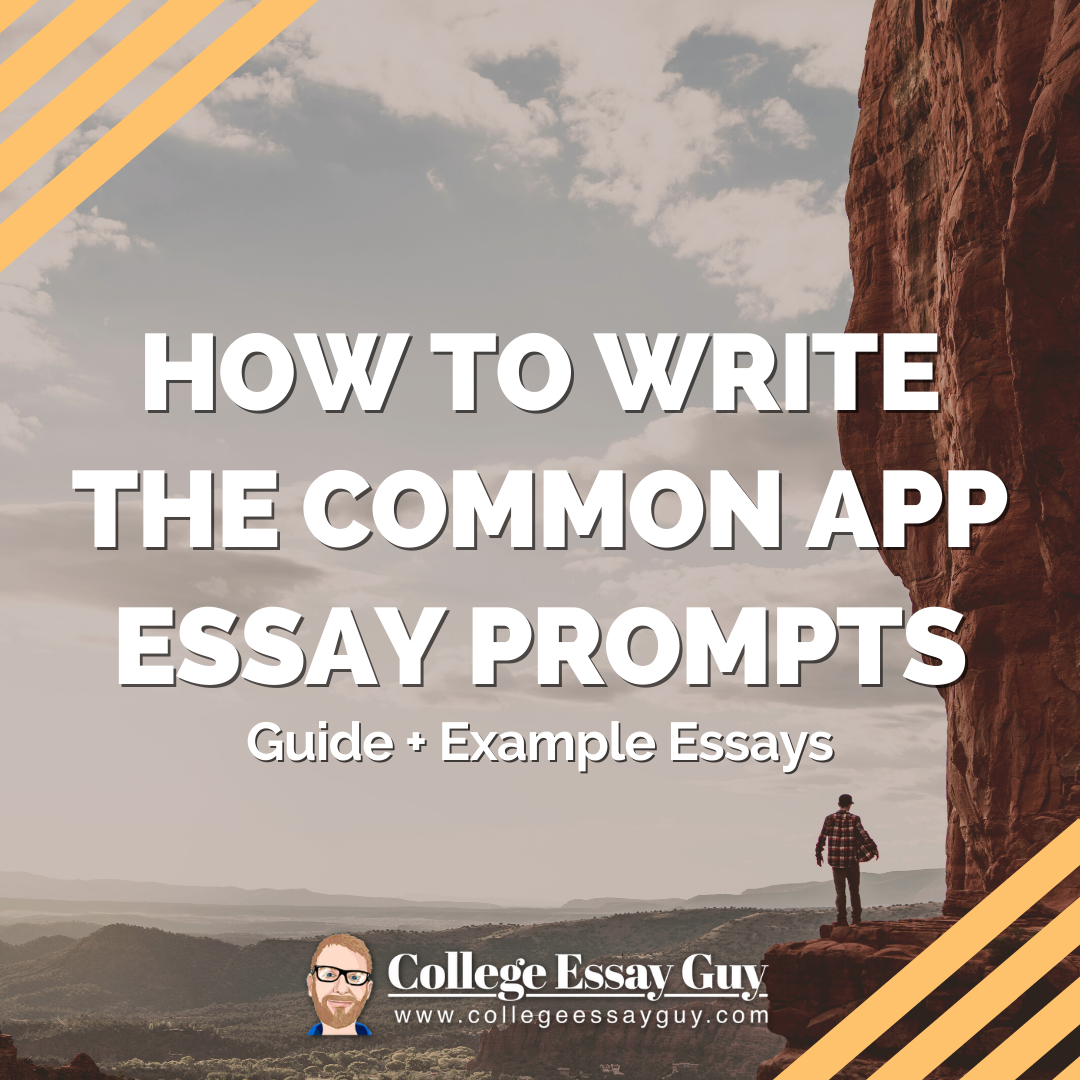The advertisement prominently features a man, likely white and with brown hair, standing on a precarious ledge of a mountain with a gray, blotchy sky overhead, indicating a gloomy, partly cloudy day. The man's back is to the viewer, and he is wearing a checkered flannel shirt and carrying a backpack, suggesting he is hiking. The rough, vertical mountain continues to rise well above his head, creating a sense of both immensity and danger. To the left of the image, there is a massive redwood tree, and the bottom part of the image shows barren, mountainous terrain. Overlaid in capital letters across the image, the text reads: "HOW TO WRITE THE COMMON APP ESSAY PROMPTS - GUIDE & EXAMPLE ESSAYS," with "College Essay Guy" and the website "www.collegeessayguy.com" at the bottom. The image sets a dramatic tone for the ad, emphasizing exploration and guidance.